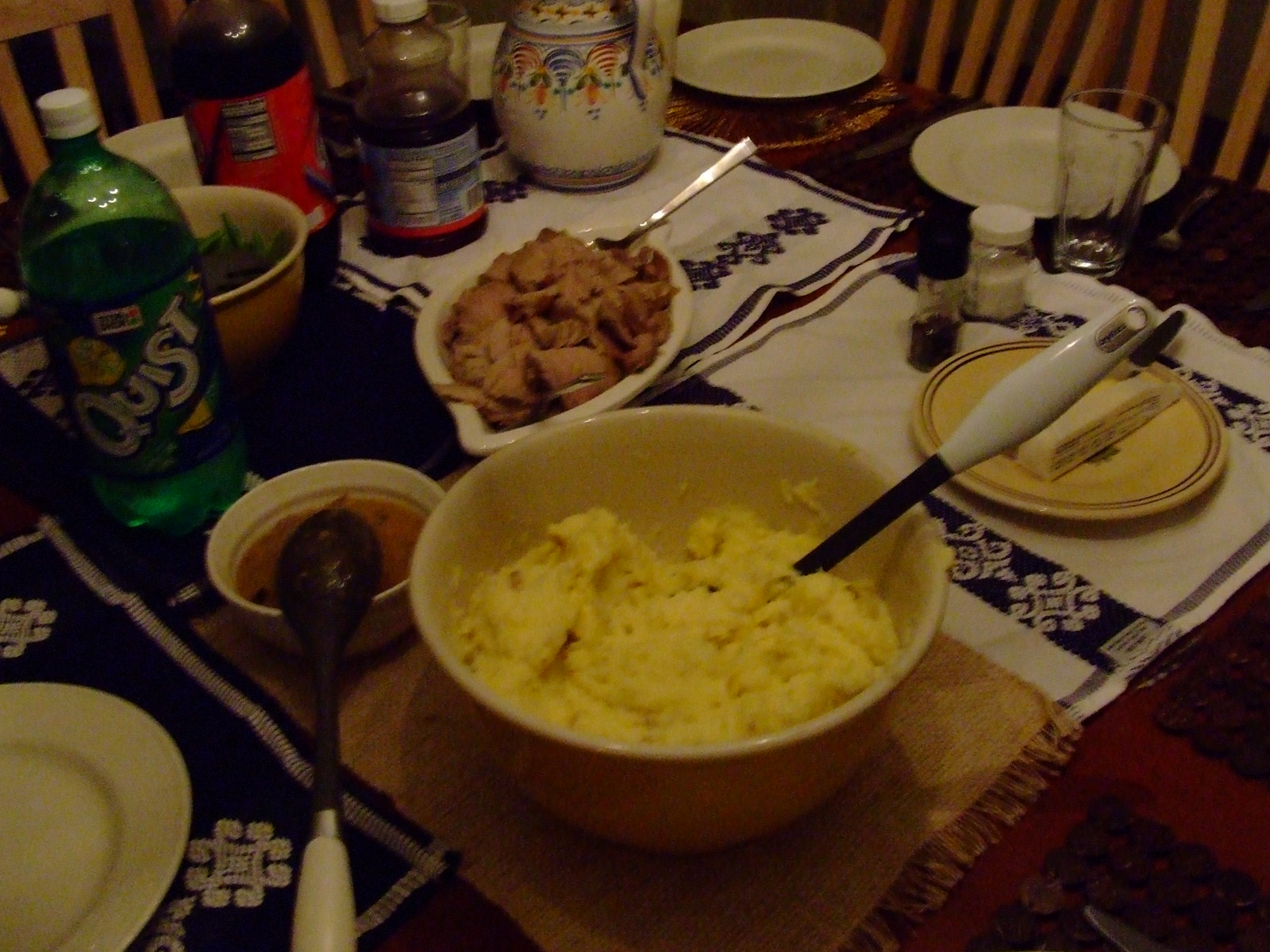The color snapshot, albeit a bit low-light and out of focus, captures an intricately set family table covered with a richly patterned tablecloth resembling Hmong embroidery designs. Dominating the foreground is a large Pyrex bowl heaped with potentially mashed potatoes, featuring a black spoon with a white handle. Adjacent to it on the left, a smaller bowl contains a brown, speckled substance, possibly gravy, with an upside-down, identical black and white spoon. Centrally located is a leaf-shaped white bowl filled with what appears to be roast beef, accompanied by a visible metal serving utensil, potentially a spoon. Closer to the viewer lies another, less visible serving utensil angled towards them. On the right, a yellow plate holds an unopened stick of butter alongside a knife with a black handle. Nearby, two plastic condiment containers, presumably for salt and pepper, one dark brown and one white, rest with their labels obscured. A clear empty glass and two white, empty dinner plates occupy the upper right section. A large white kettle with blue, red, orange, and green curved designs sits amidst a glass jug of dark purple juice, likely grape, and a red-labeled bottle of dark soda turned away from view. An orange bowl with a green interior design contains what appears to be blue chips, resting near a distinct green bottle of Quist soda, emblazoned with a lemon-lime logo similar to Sprite. The lower left side features an empty white plate on a blue cloth, contrasting with a red cloth on the lower right and white cloths adorned with blue details towards the back center. Lastly, there are tall slat-back chairs encircling the table, establishing the setting as a warm and inviting family gathering.